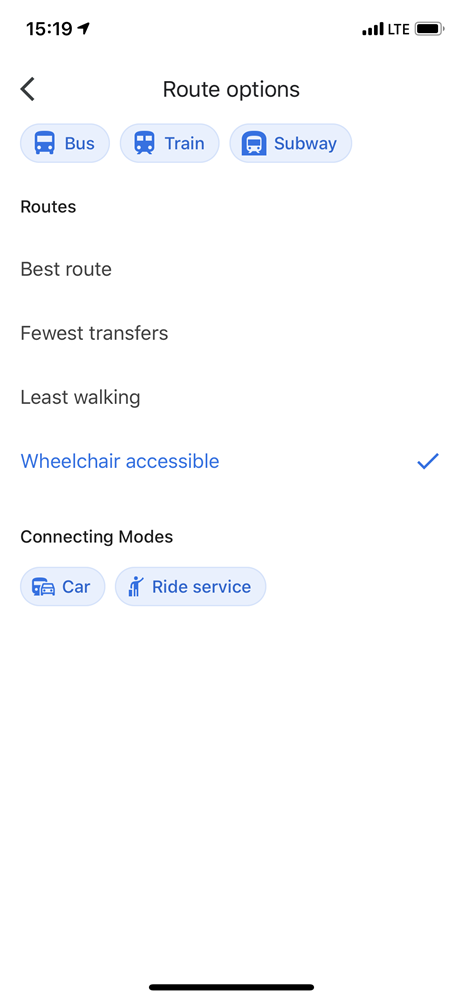In the upper left corner, the time is displayed as 15:19, accompanied by a small arrow diagonally pointing upward. To the right, there are four ascending bars that indicate signal strength, followed by the acronym LTE in uppercase letters, and an almost full battery icon.

Directly below this status bar, the text "Route Options" is displayed, with an arrow pointing left. Three blue ovals are lined up beneath, each containing different icons: the first depicts the front of a bus with the word "Bus" next to it, the second shows an image of a train, and the third features a subway icon, characterized by a square-shaped front with a rectangular window cutout.

Below these ovals, the word "Routes" is presented in black text. Approximately two inches below, there are sequential options listed: "Best Route", "Fewest Transfers", "Least Walking", and "Wheelchair Accessible", the last of which is highlighted in blue with a blue checkmark to the right.

Further down, in black text, it says "Connecting Modes". This is followed by two blue circles: the first contains an image of a car alongside the word "Car", while the second shows a person holding up their thumb with the label "Ride Service".